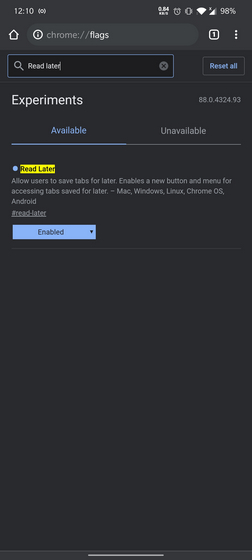The image shows a screenshot of a smartphone's display, capturing the Chrome browser with the URL `chrome://flags` entered in the search bar. The device indicates strong connectivity with full signal bars and a battery level of 96%. Below the URL, a secondary search bar contains the term "Read Later," accompanied by a small "X" icon for clearing the search.

The screen is divided into sections labeled "Experiments," "Available," and "Unavailable." The "Available" section is highlighted in blue, contrasting with the gray "Unavailable" section. A feature titled "Read Later" is prominently displayed within a yellow rectangle featuring black text. This feature description – "Allow users to save tabs for later. It enables a new button and a menu for accessing tabs saved for later." – spans multiple lines and indicates compatibility across Mac, Windows, Linux, Chrome OS, and Android platforms. The phrase "Read Later" is underlined, suggesting a hyperlink or important annotation.

Adjacent to the feature description is a blue button labeled "Enabled," signifying that the "Read Later" function is active. This button has an embedded pull-down menu. The interface's background is predominantly black, with various text and button elements in shades of gray, white, blue, and yellow. The overall visual theme emphasizes dark tones, with black being the most dominant color, underscored by lighter highlights and colored accents to differentiate interactive elements and text.